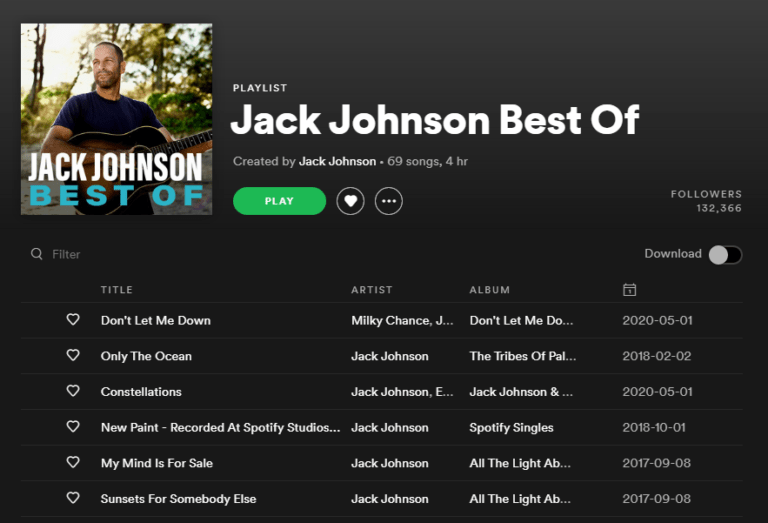The image features a dark gray interface displaying a music playlist. On the left side, there is an album cover showing a man with a beard stubble, standing outdoors with trees and sky in the background. He is wearing a navy blue short-sleeved shirt and holding a brown acoustic guitar. The album cover reads "Jack Johnson Best Of."

To the right of the album cover, the playlist details are displayed. The playlist is titled "Playlist: Jack Johnson Best Of," created by Jack Johnson. It contains 69 songs. Below the playlist title, there are icons: a green play button, a circle with a heart inside, a circle with an ellipsis, and a toggle switch labeled "Download," which is turned to the left. The playlist has "Followers: 100 and something thousand," though the exact number is blurry.

Under these details, there are four columns labeled "Title," "Artist," "Album," and "Date." The first row lists the song "Don't Let Me Down" by Milky Chance from the album "Don't Let Me Down," dated 2020-06-05. The second row lists the song "Only The Ocean" by Jack Johnson.